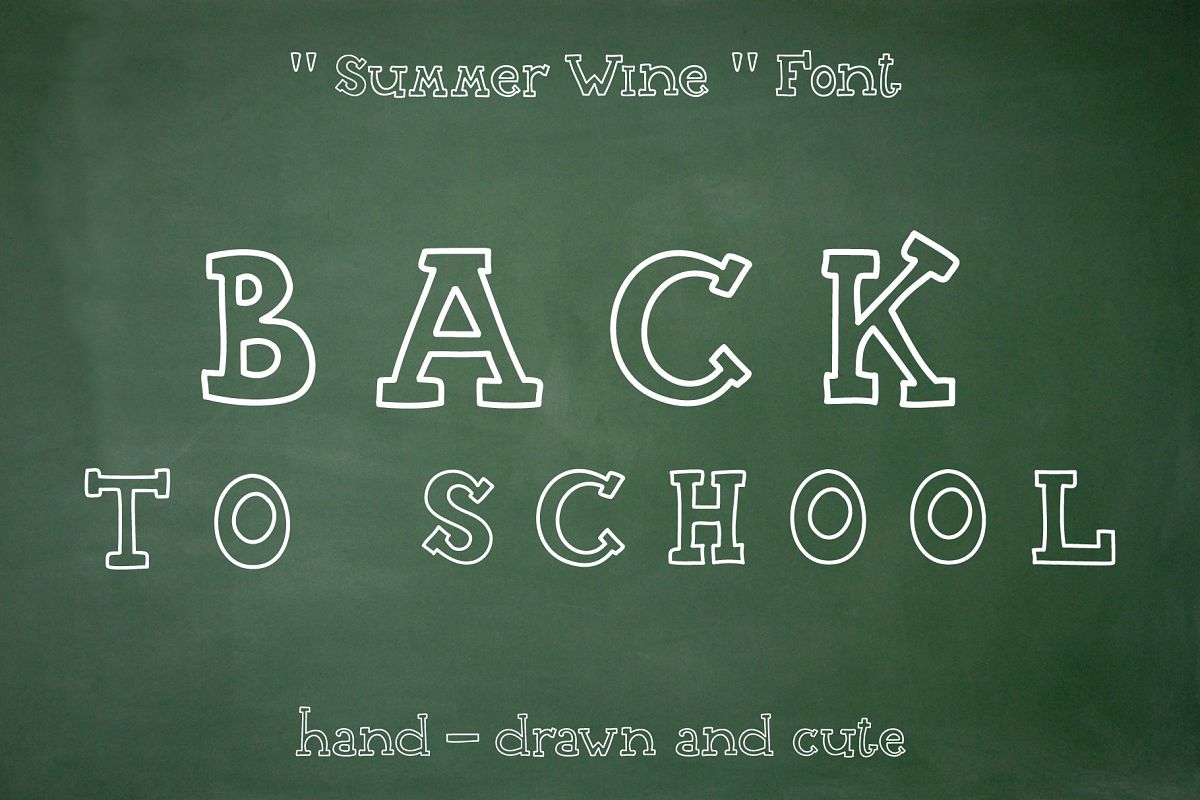The image features a solid dark gray background with a subtle marble texture, incorporating a mix of gray and white hues. At the top, the phrase "summer wine" is prominently displayed in a stylistic font, enclosed within quotation marks. Centered in the image are large, blocky letters spelling out "BACK TO SCHOOL" in all capitals. The word "BACK" appears slightly larger than "TO SCHOOL," and each letter is outlined in white. Below this, in a smaller, hand-drawn and cute style, are the words "hand-drawn" and "cute" separated by dashes. The overall composition has a cohesive and visually appealing design, merging both the refined marble texture and the playful handwritten elements.